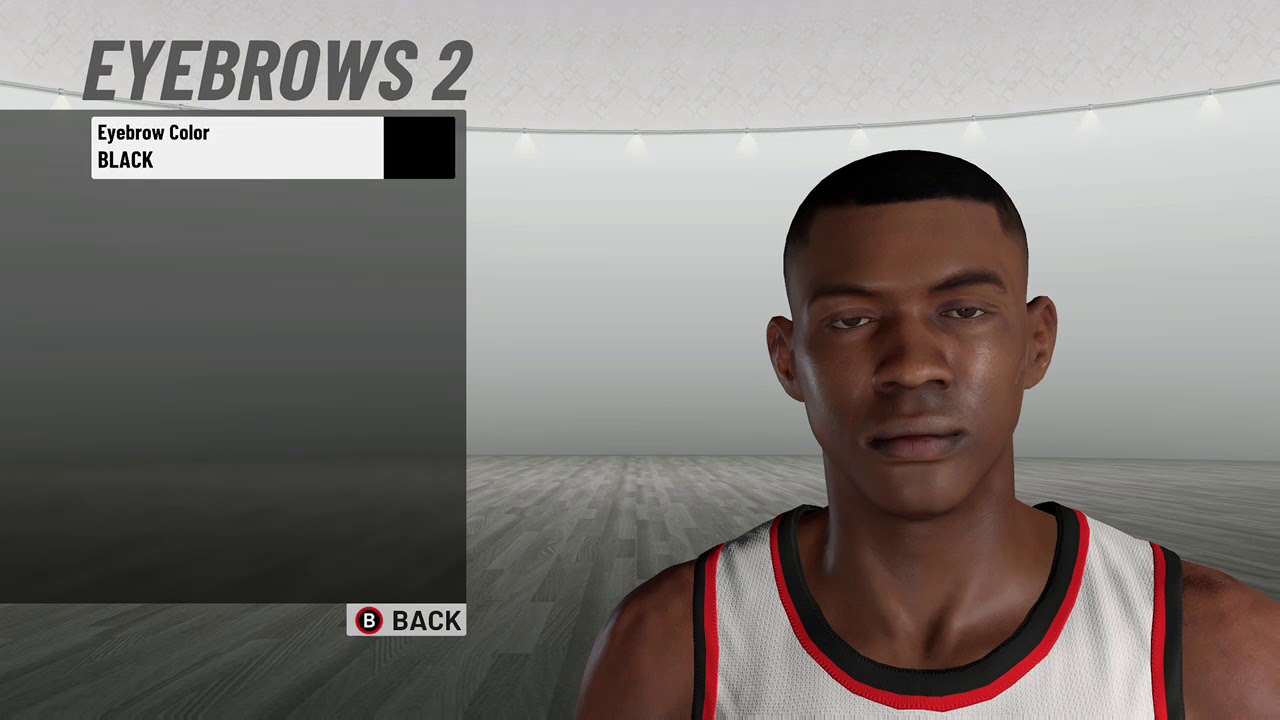Caption: In this detailed digital illustration, a young Black man is portrayed wearing a stylish basketball vest, suggesting he is either an athlete or a character from a sports-focused website where users can create their own avatars. The background is a meticulously designed, rounded room with a smooth, pale grey curved wall adorned with downlighters at its edge, setting a modern and atmospheric scene. The ceiling is a crisp white, adding to the clean look of the space. Grey wood effect tiles extend from the lower part of the man's shoulder down to the base of the curved wall, providing a textured contrast.

In the upper left corner of the image, dark grey capital letters spell out "EYEBROWS" followed by the number 2, indicating an editable feature. Just below, a dark grey opaque block appears, containing options to further customize the avatar. Within this block, a white rectangle with the text "Eyebrow color: BLACK" and an adjacent black square suggest further personalization choices. At the bottom of this block is a distinct grey button with a circular emblem, featuring a red and black background with a prominent white letter "B" and the word "BACK," likely facilitating navigation back to a previous menu. These details allude to an interactive and customizable user interface designed for avatar creation.